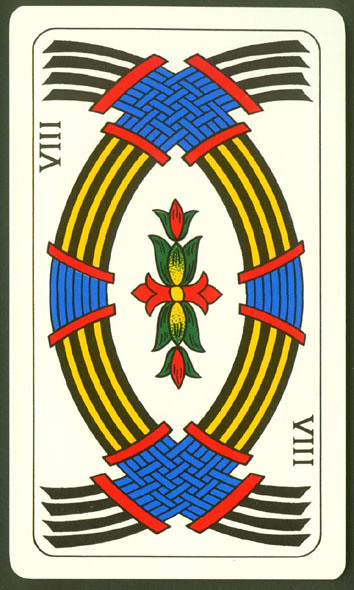This detailed photograph captures a tarot card adorned with intricate symbolism and vibrant colors. The card features the Roman numeral VIII prominently in both the upper left and lower right corners, indicated by a V followed by three vertical lines. At the top and bottom edges of the card, we observe crisscrossed blue lines that intersect and create a meshed pattern.

Extending from these blue intersections, black and white stripes fan out towards the corners of the card, specifically in the upper right, upper left, lower right, and lower left sections. The card's central focal point is a floral design, vividly depicted with lush green leaves at the top and bottom. The flower's core is a rich red adorned with delicate plumes, while additional patches of gold, green, and red embellish its center.

The card's background is predominantly white, yet it is divided by striking black and yellow stripes that alternate in both the upper and lower halves. These stripes echo the theme of contrast and duality present throughout the design. Overall, this tarot card is a harmonious blend of repeating colors, patterns, and symbolic elements that invite deeper contemplation and interpretation.